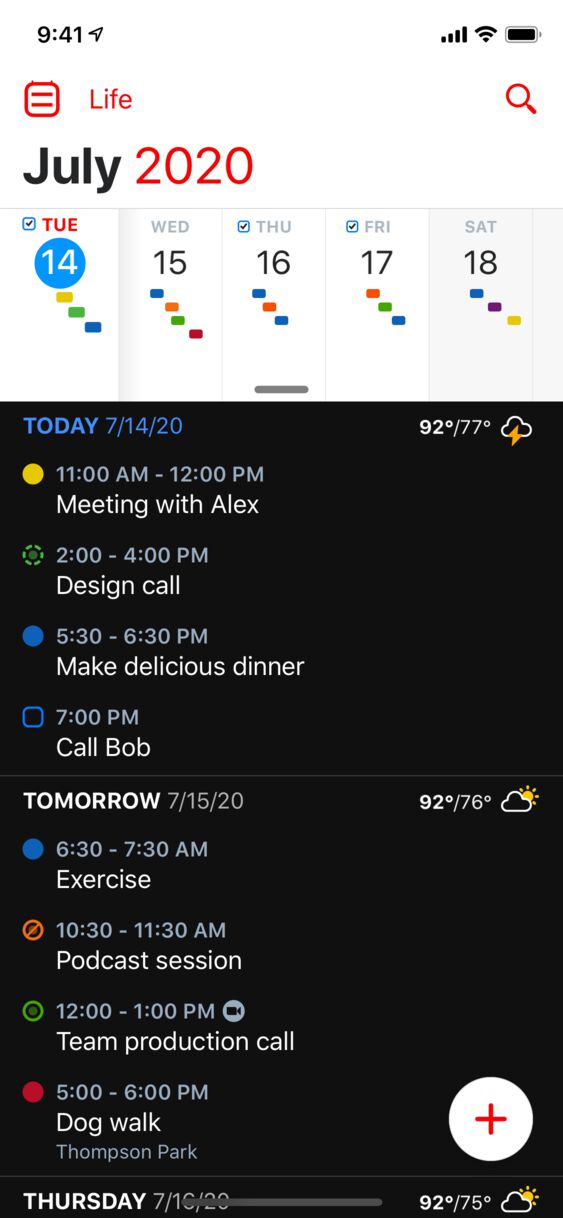This image is a screen capture from a cell phone displaying a scheduling app. The time on the phone is 9:41, and it shows a fully charged battery, strong Wi-Fi connectivity, and a full cellular signal. The app is set to July 2020, specifically Tuesday, July 14th, and presents a detailed list of scheduled events alongside a reminder.

For today, the temperature is indicated as a high of 92°F and a low of 77°F. The schedule includes:
- A meeting with Alex from 11:00 AM to 12:00 PM.
- A design call from 2:00 PM to 4:00 PM.
- A task to make a delicious dinner from 5:30 PM to 6:30 PM.
- A reminder to call Bob at 7:00 PM.

Additionally, the app shows a preview of the events scheduled for tomorrow:
- Exercise from 6:30 AM to 7:30 AM.
- A podcast session from 10:30 AM to 11:30 AM.
- A team production call from 12:00 PM to 1:00 PM.
- A dog walk at Thompson Park from 5:00 PM to 6:00 PM.

The interface also allows scrolling down to view the schedule for Thursday and the remainder of the week, ensuring comprehensive planning and organization.